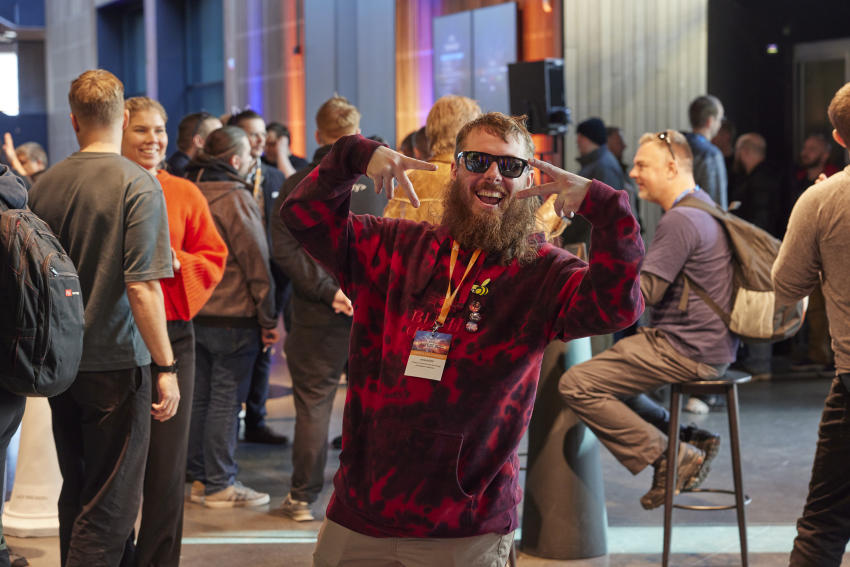This photograph captures a bustling scene inside a public setting, possibly a convention center or building lobby, teeming with people. Dominating the center of the frame is a bearded man with orangish-brown hair, a mustache, and a large beard. He radiates excitement and joy, smiling broadly while holding up two peace signs. His attire is striking - a vibrant tie-dye hoodie in various shades of red and dark red, paired with khaki pants and black sunglasses. An orange lanyard with a tag dangles around his neck.

Behind him, the ambiance is lively and colorful. The background features walls in different colors, such as blue, and a white curtain illuminated by purple and orange lights. A diverse crowd mills around, socializing and chatting. Notably, a man in a gray t-shirt and dark pants speaks to a blonde woman in an orange top and black pants, while further back, a man with a backpack sits on a stool, and a girl in an orange sweatshirt smiles, contributing to the cheerful atmosphere. The photograph vividly depicts a moment of communal joy and interaction, centered around the bearded man's playful and spirited pose.